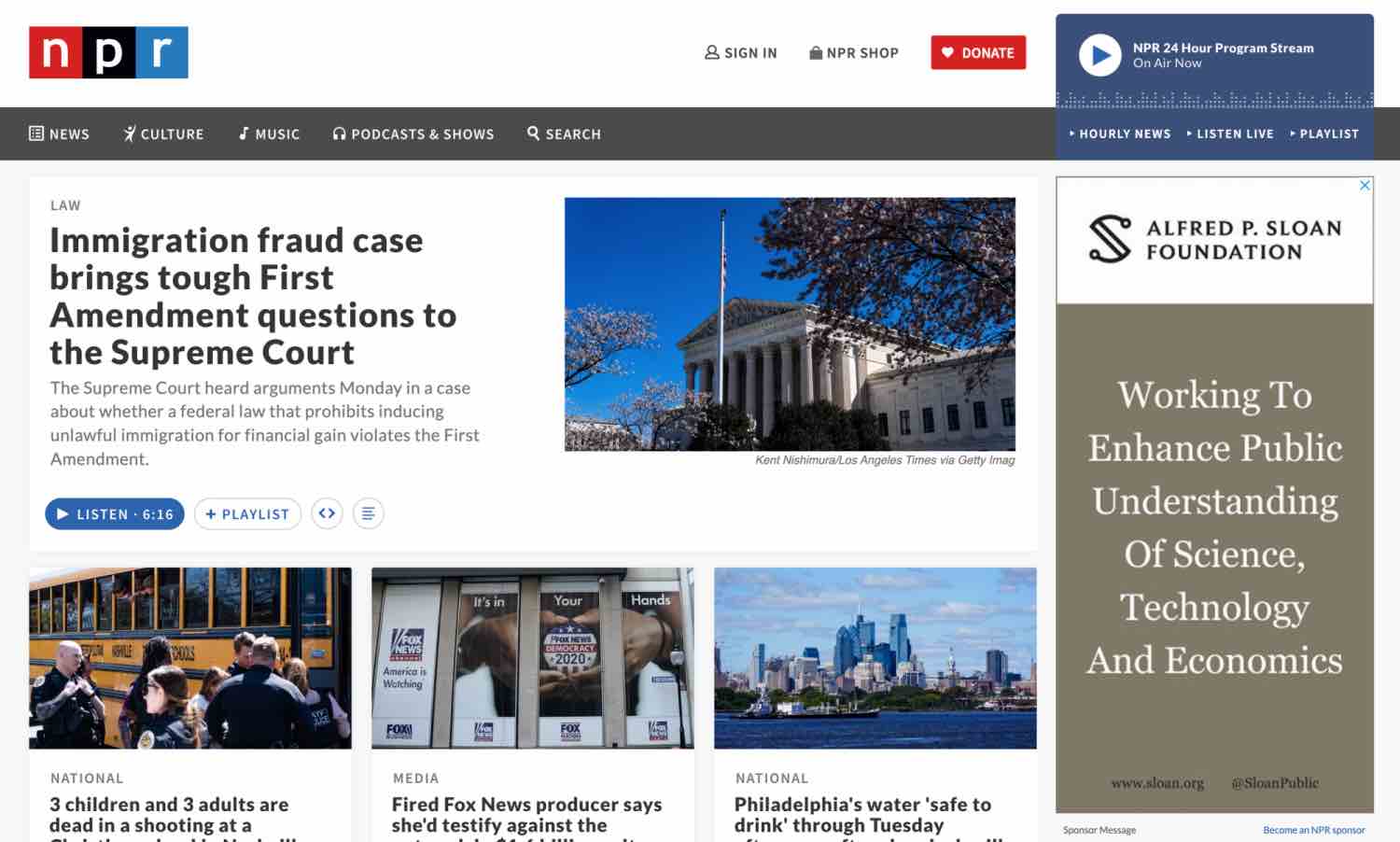Screenshot of NPR's Homepage: 

In the upper left-hand corner, there are three small squares. The left square is red with a lowercase white 'n', the middle square is black with a lowercase white 'p', and the right square is blue with a lowercase white 'r'. 

On the right side of the page, there's a button labeled "Sign In" and another button for the "NPR Shop". Additionally, there is a prominent red "Donate" button featuring a white heart symbol, with the word "Donate" in white. 

In the top center of the page, there is a blue rectangle with a white play icon inside. To its right, it says "NPR 24-Hour Program Stream" in white. 

Below this is a dark gray menu bar, with each menu item written in white. The menu options include News, Culture, Music, Podcasts & Shows, and Search. Towards the right end, there are dropdown options for Hourly News, Listen Live, and Playlist. 

The background below these elements is white. On the left-hand side, there is a headline in bold black text that reads, "Immigration Fraud Case Brings Tough First Amendment Questions to the Supreme Court." A brief paragraph below the headline provides more context. Beneath this paragraph, there is a blue "Listen" button and a white "Playlist" button. 

To the right of this headline and its accompanying text, there are three image squares. The top lines of the headlines beneath these images are partially visible.